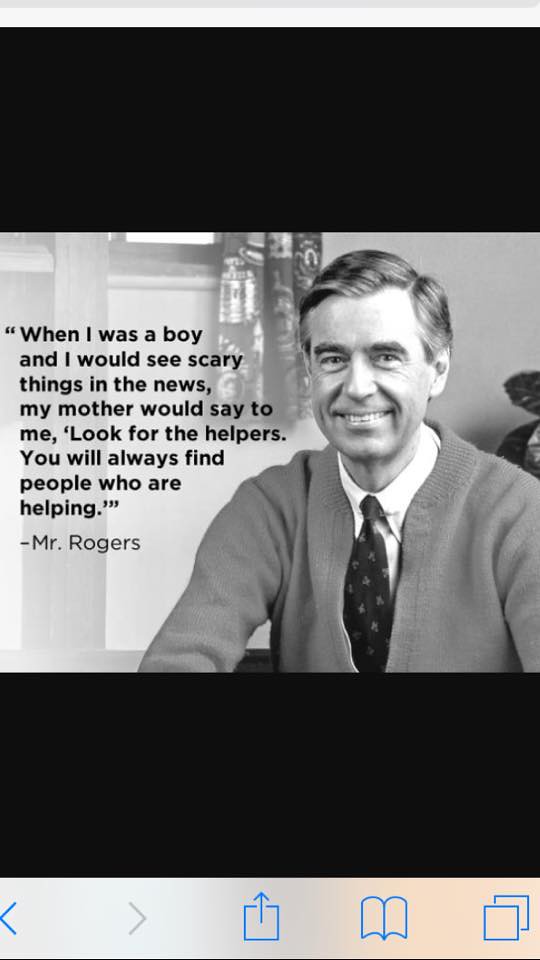This is a detailed screenshot from an iPhone or possibly an iPad, displaying the iOS Safari browser interface. At the bottom of the screenshot, typical browser icons are visible, including back and forward arrows, a download button, a bookmarks button, and icons to open or switch between tabs.

The central focus of the screenshot is a black-and-white meme featuring a smiling Mr. Rogers. He is dressed in his iconic sweater and tie, sitting in what appears to be the familiar setting of his TV show, with neatly combed hair and a room backdrop featuring a wall, curtains, and possibly a potted plant. To the left of his image, there is a heartfelt quote attributed to Mr. Rogers: "When I was a boy and I would see scary things in the news, my mother would say to me, 'Look for the helpers. You will always find people who are helping.'" The meme is bordered by black bars at the top and bottom, framing the quote and image nicely.